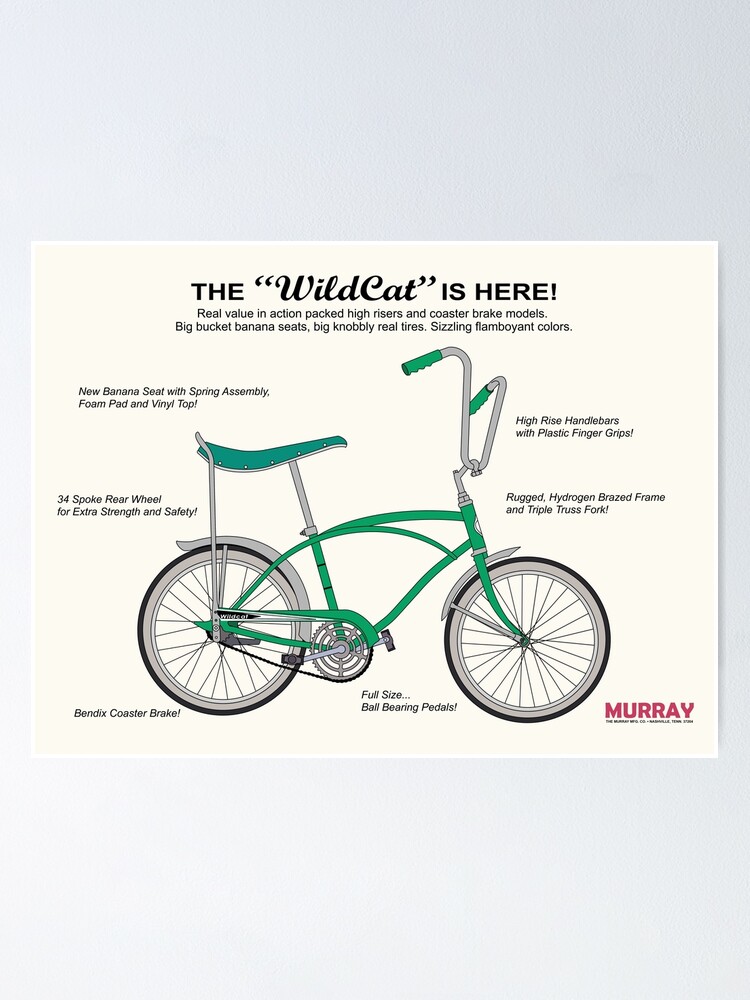The image features an off-white square section centered on a light or bluish-gray background. In the upper portion of this off-white section, black text declares "The Wildcat is here" in a large cursive font. Below it, additional text boasts features such as "real value in action-packed high risers and coaster brake models," "big bucket banana seats," "big knobby wheel tires," and "sizzling flamboyant colors." At the heart of the image, a detailed drawing or artist's rendering of a green bicycle is displayed. The bike is meticulously labeled, showcasing its distinctive features: green handlebar tips, a green long banana seat, silver lower handlebars, and silver racks. The bicycle's fenders are gray, its tires are a mix of white, gray, and black, and it comes equipped with full-size ball-bearing pedals. Surrounding the bike, various informative labels describe components such as the "new banana seat with spring assembly," "foam-padded vinyl top," "34-spoke rear wheel for extra strength and safety," and "rugged hydrogen bronze braced frame with double truss fork." In the bottom right corner, the brand name "Murray" is prominently displayed in red capital letters, accompanied by smaller, less legible text beneath it.